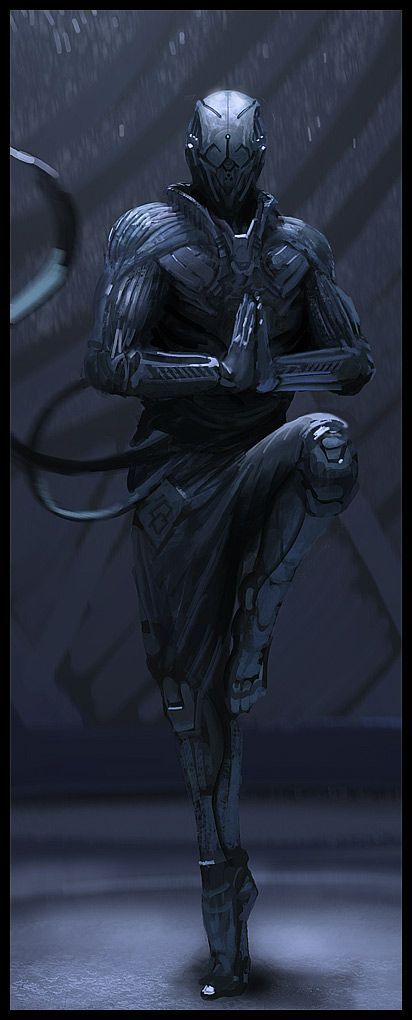The image is a vertically long artistic depiction of a humanoid science fiction character, standing in a martial arts pose on one foot, specifically on their tippy toes. The overall color palette is dark grey and black, with a matching grey background streaked with black. The character is clad in a sleek, muscular suit that emphasizes the silhouette of their deltoids. They have their other leg drawn up, with the knee pointing outward and the foot resting near the standing knee. Their arms are bent at the wrists with their hands clasped together directly in front of their chest, palms facing each other, and fingers pointing upward, almost as if in prayer. Instead of a human head, the character has a featureless mask or some indiscernible element. Black wires protrude from the left side of their body, swirling outward and off the image. Additionally, the character appears to have a tail or tentacle-like appendage at the front. The overall theme is fantasy, with the character exuding an enigmatic, possibly dark superhero or villain vibe.